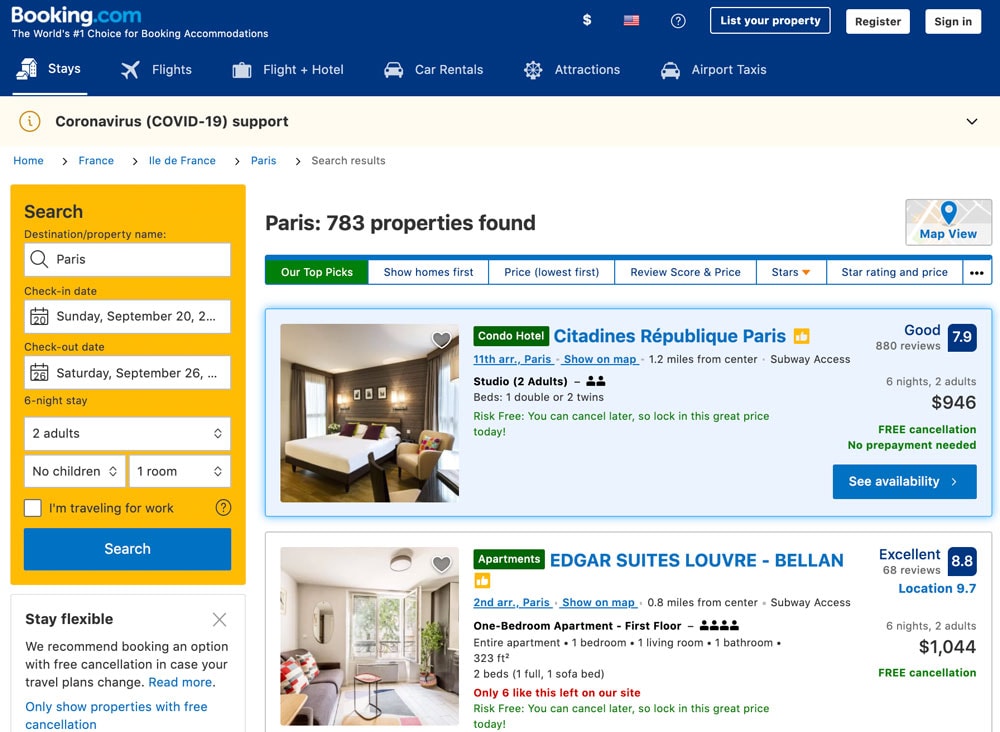This screenshot captures an advertisement for Booking.com, showcasing its platform for booking various accommodations, similar to other apartment rental applications. In the top left corner, the Booking.com logo is prominently displayed, with the tagline "The world's number one choice for booking accommodations" just below it. Adjacent to these elements are icons for currency (dollar sign), language (American flag), and help (question mark), along with three buttons labeled: "List your property", "Register", and "Sign in".

Directly below these features, six horizontal tabs allow users to navigate different sections of the website: "Stays", "Flights", "Flight + Hotel", "Car Rentals", "Attractions", and "Airport Taxis". A banner notice offers COVID-19 support, highlighting the platform's dedication to traveler safety.

On the left side of the page, a search menu indicates that the user has queried for accommodations in Paris from September 20th to September 26th, for two adults in one room. The search results are displayed on the right side of the screen. The first recommendation is the Citadines République Paris, a condo hotel studio rated as "Good" with a score of 7.9, priced at $946. Below that is Edgar Suites Louvre - Belan, an apartment rated as "Excellent" with a score of 8.8, available for $1044.